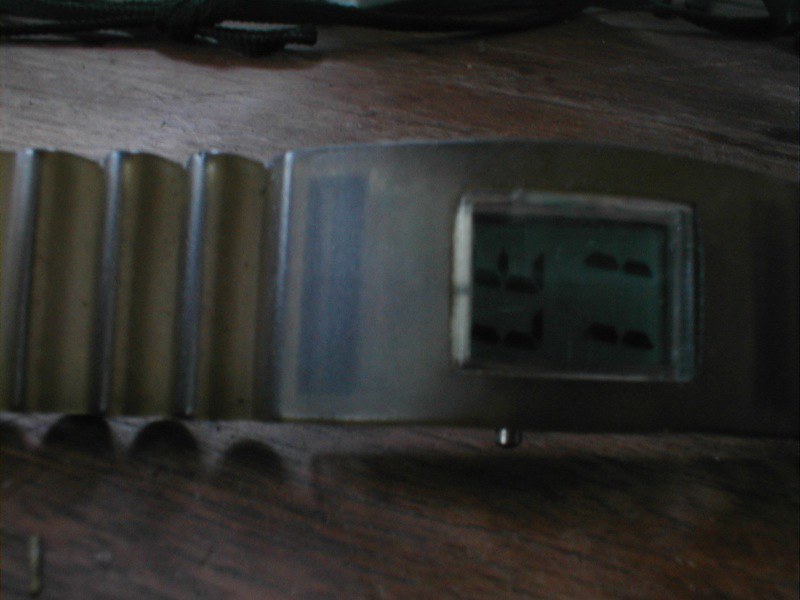In this dark, atmospheric scene, an old and worn digital watch with a rectangular face lies horizontally on a dark brown wooden table. The watch, made of a tarnished brass or gold-colored metal, displays the numbers "11" at the top and "37" at the bottom, which are somewhat difficult to read due to the image's poor lighting. The wristband is elaborately designed with grooves and divots, but looks uncomfortable due to its bumpy texture. Additionally, there are several wires visible at the top of the shot, adding to the cluttered and aged aesthetic of the setting.